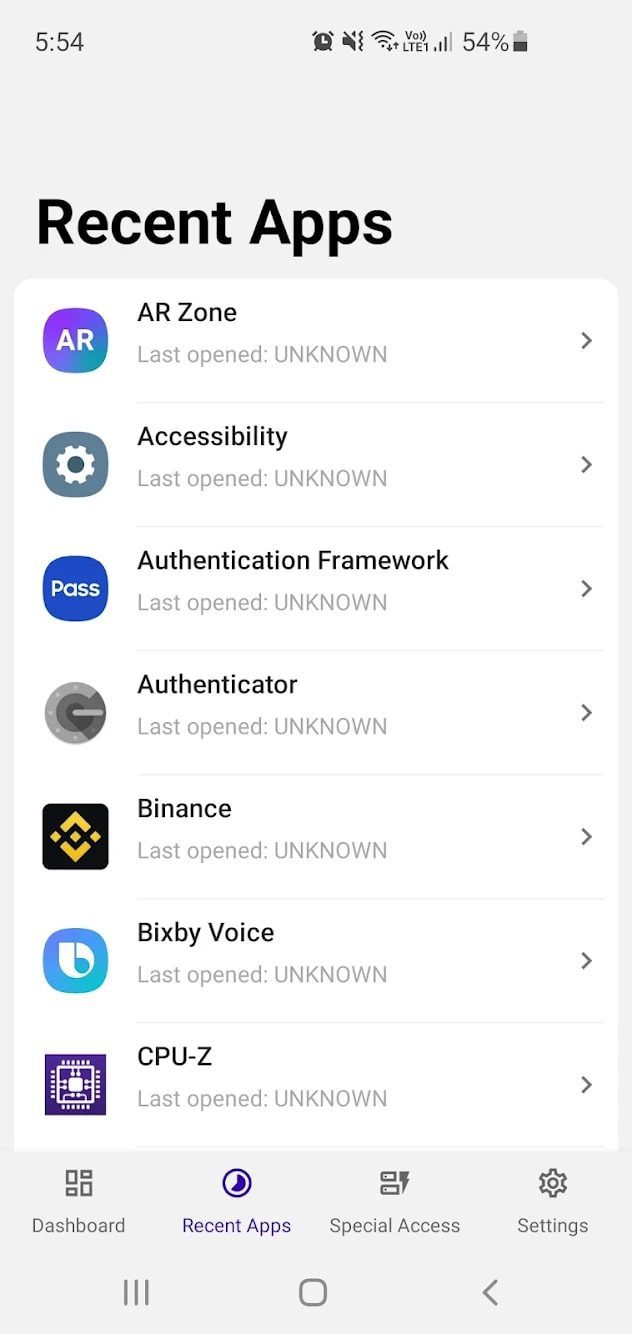The image shows a smartphone screen with the number "554" displayed on the left. On the main portion of the screen, the header "Recent Apps" is prominently written in bold black letters, with "Recent" and "Apps" both capitalized. Below this header, a list of applications is visible. Each application name is written in bold black text and is accompanied by its respective icon on the left. The listed applications, from top to bottom, are: 

1. AR Zone - Icon: A purple and blue logo with "AR" in white
2. Accessibility
3. Authentication Framework
4. Authenticator
5. Binance
6. Bixby Voice
7. CPU-Z

Beneath each application name, in light gray text, it says "Last Opened: UNKNOWN," with "UNKNOWN" in all capital letters. At the very bottom of the screen, a navigation bar contains options written in black text: "Dashboard," "Recent Apps," "Special Access," and "Settings," listed from left to right.